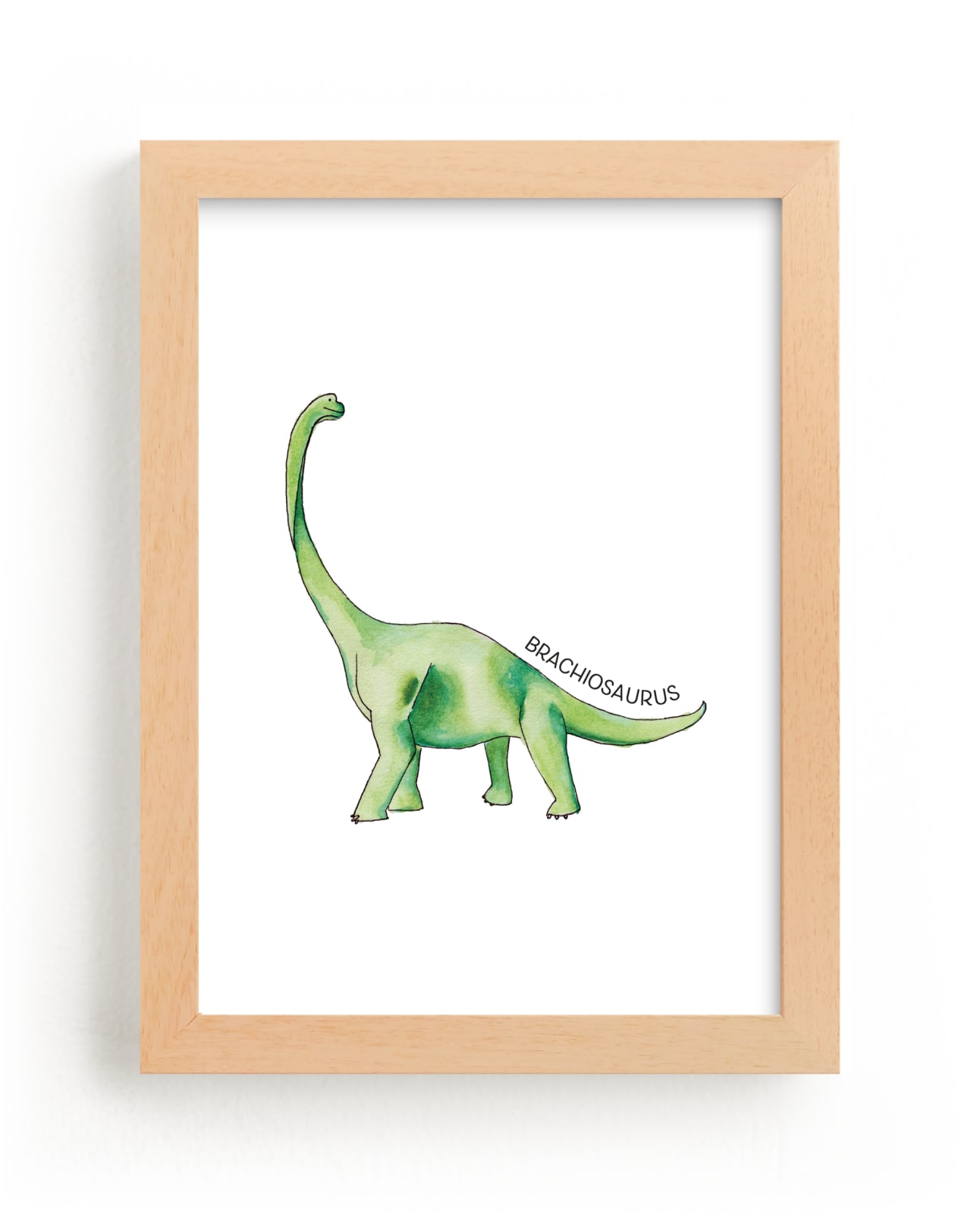The image captures a framed illustration of a green Brachiosaurus dinosaur on a white background. The light-colored wooden frame has no matting and is mounted on a white wall, casting a shadow to the left, indicating a light source from the upper right. The Brachiosaurus, depicted in shades of dark and light green, has a small head, a long neck, and is looking behind itself. The dinosaur stands on four legs with noticeably sharp claws. Above its tail is the label "BRACHIOSAURUS" in all capitalized gray letters. The illustration appears to be hand-drawn and watercolored, set upon a blank white paper.